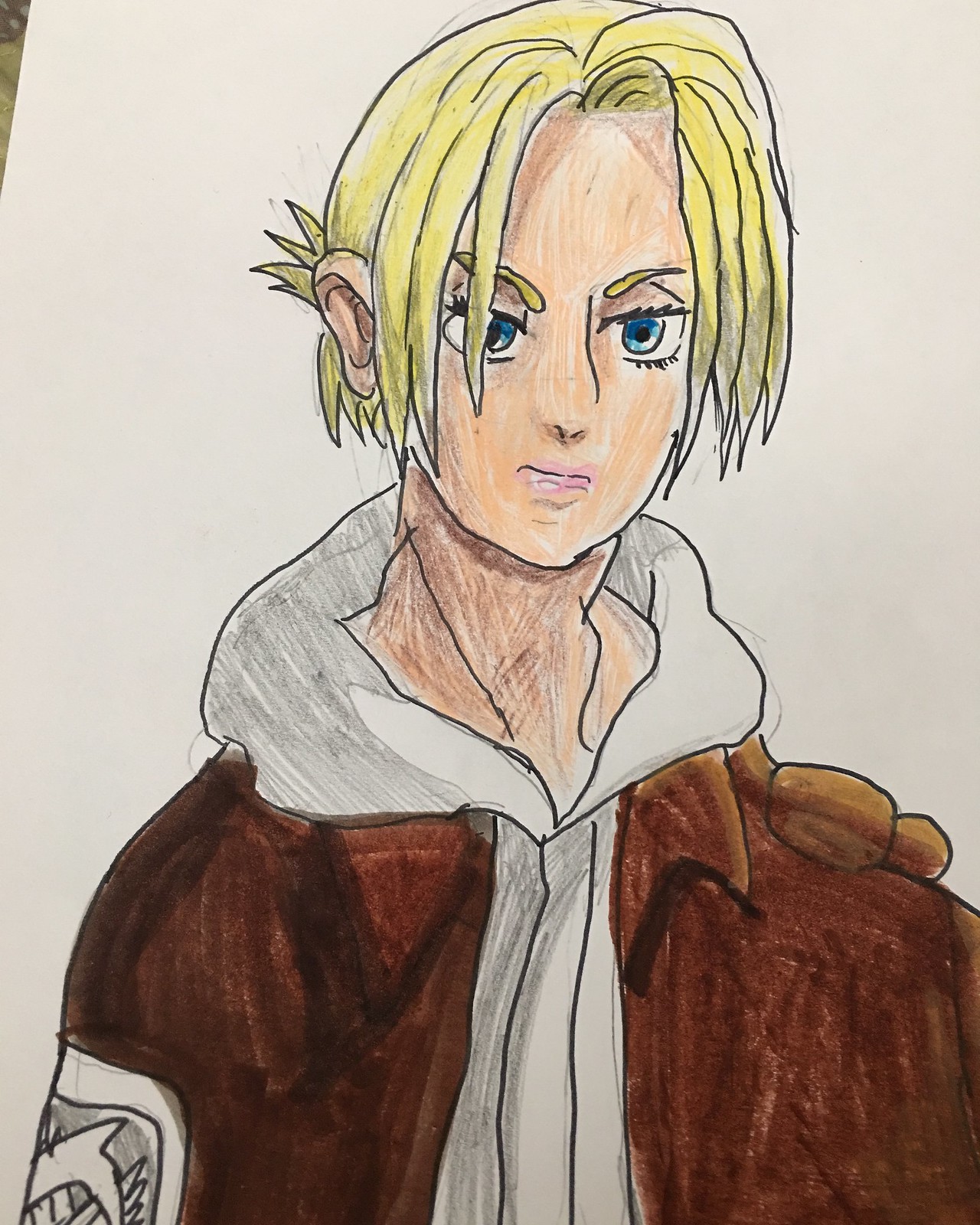In this vibrant close-up artwork, the medium used appears to be colored pencils. The illustration showcases a detailed depiction of an anime character, portrayed as a fair-skinned young man. His wide, oversized blue eyes convey a sense of intensity, complemented by his long, blonde bangs that partially frame his face. He is dressed in a brown bomber jacket layered over a light gray and white hoodie, meticulously colored to highlight the textures and folds. The artwork is outlined with precision in black pencil, while the skin tones are rendered in soft flesh hues and the hair is vividly colored in yellow, giving it a lifelike sheen. The character is portrayed from the chest up, gazing forward with a serious and contemplative expression, capturing a moment of stillness and depth.